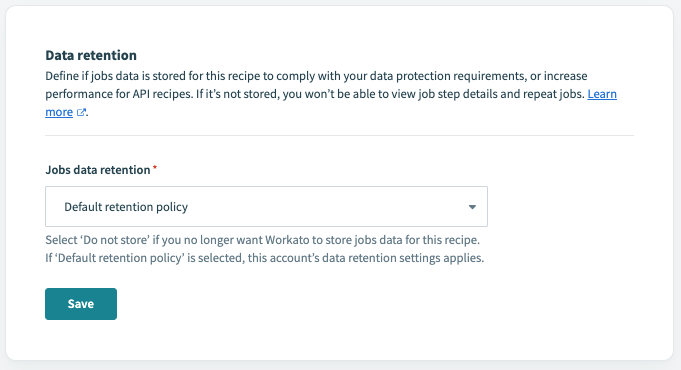Close-up of a user interface from a website featuring a data retention settings window. The background has a faint gray border around the edges while the main content area is white. At the top, bold black text states "Data Retention". Below this, in smaller, regular black font, it reads: "Define if job data is stored for this recipe to comply with your data protection requirements or increase performance for API recipes. If it’s not stored, you won’t be able to view your job step details and repeat jobs." 

An underlined blue "Learn more" link follows this text. Underneath, a faint gray line separates the sections. 

Next, bold black text reads "Job Data Retention" accompanied by a red star indicating a mandatory field. Below it is a dropdown menu labeled "Default retention policy", suggesting that the retention settings can be changed. In gray text, it reads: "Select ‘Do not store’ if you no longer want Workato to store job data for this recipe. If 'Default retention policy' is selected, this account's data retention settings apply."

At the bottom of the window, a turquoise blue button labeled "Save" in white font is present for saving the settings.